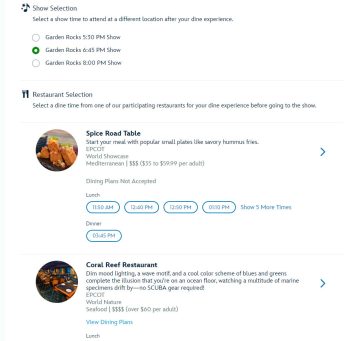This screenshot, presented against a white background, is notably out of focus and somewhat blurry. At the top, it features black text alongside a gray icon, possibly a music note, that reads "Show Selection." Below this header is a prompt instructing users to select a show time to attend after their dining experience. Three show time options are listed:

1. "Garden Rocks" at 5:10 PM
2. "Garden Rocks" at either 6:45 PM or 6:15 PM (the exact time is unclear due to the blurriness)
3. "Garden Rocks" at 8:00 PM

The middle option is selected, indicated by a green radio button to the left.

Further down, there is a gray knife and fork icon followed by the text "Restaurant Selection." The section invites users to "Select a Dine Time," but the details are too blurry to decipher.

In the next section, a circle on the left displays stacked beige-colored meat, suggesting the dish offered. The accompanying text reads "Spice Road Table," inviting users to select a meal featuring popular small plates. However, the text remains largely illegible. To the far right, there is a blue right-arrow icon.

Beneath it, the words "Dining" appear, accompanied by a note that dining something (possibly reservations) is not accepted. Under "Lunch," four oval blue buttons display selectable times, with an option to "Show 5 more times" on the far right in blue. For "Dinner," only one available time is listed in an oval button with no option to select more times.

The last section includes a round image on the left, depicting a counter in a restaurant or trays with food. To the right, it reads "Coral Reef Restaurant," followed by "View Dining Plans" in blue text. A blue right-arrow icon is positioned on the far right.